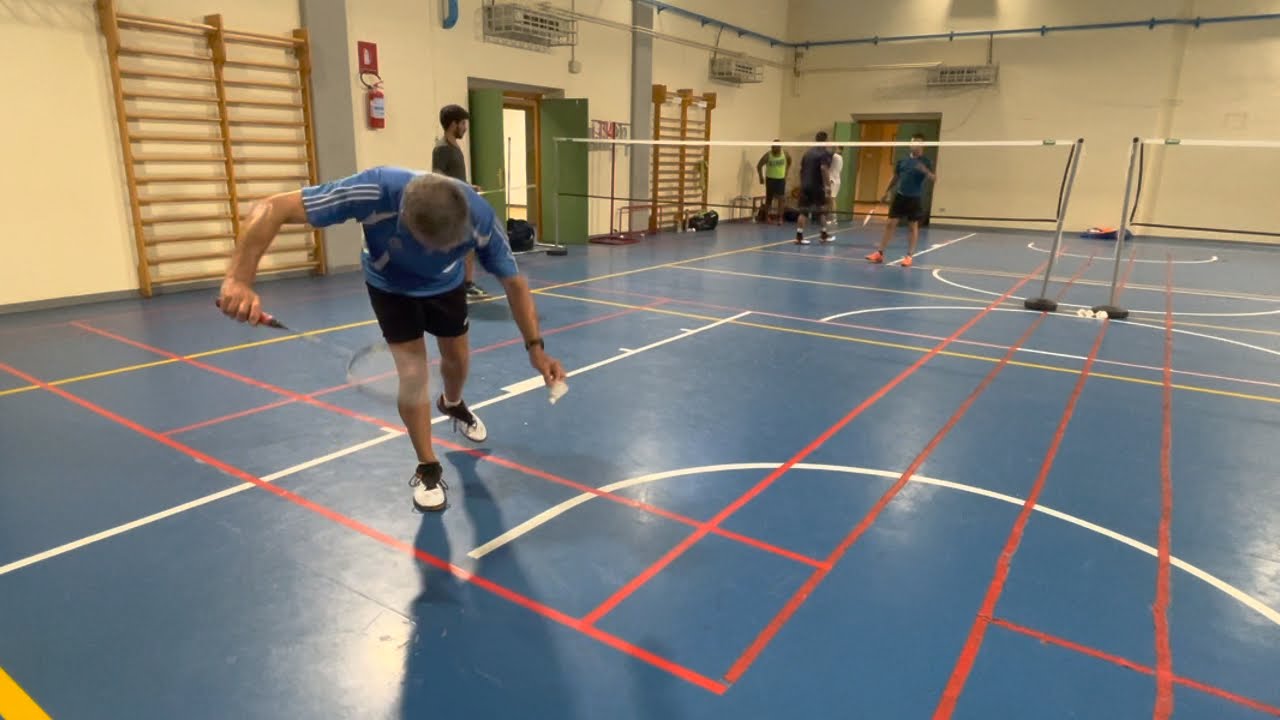The image depicts an indoor gymnasium with a blue reflective floor marked by red, white, yellow, and some purple lines, indicating various sports courts. Dominating the center are two adjacent nets, likely set up for badminton given the context. Prominently, in the foreground, a man in a blue jersey with white detailing, black shorts, and white sneakers with black laces is poised to serve. He is bent slightly forward, facing the camera, and holding a tennis racket in motion, serving a badminton birdie. His dynamic movement makes the racket appear blurry. Behind the nets, four other players await on the opposing court side, signaling an ongoing game. The gym's walls are white, and there are wooden rings mounted around a door on one side of the nets. Additionally, an open double door can be seen in the top background of the image, adding depth to the scene. The lighting is bright, illuminating the entire space effectively for indoor sports activities.